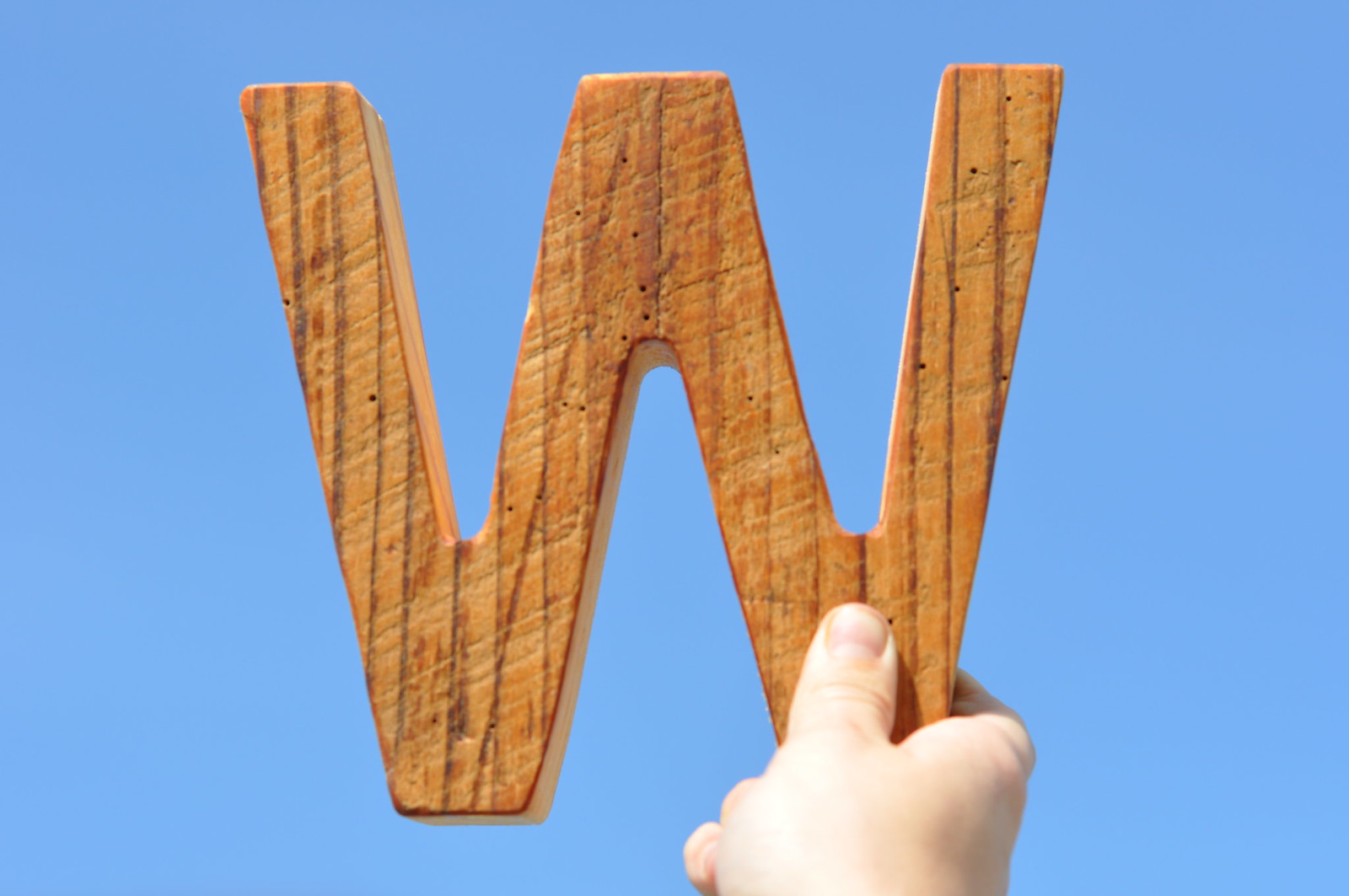The image depicts a right hand holding a large, wooden W in front of a light blue background, possibly the sky. The hand, visible from the top down to where it extends off the bottom right corner of the image, grasps the W by its bottom end, near the second V shape, with the thumb prominently positioned over this section. The fingers wrap around the wooden structure, contributing to the sense of scale indicating that the W is about the size of two spread out hands. The wooden W, centered in the image, exhibits a brown hue with vertical, darker striations and a slightly grainy texture, confirming its wooden material. The construction of the W appears to resemble two V shapes joined together, with a noticeable seam at the middle top where the Vs converge. The background's light blue color fades slightly lighter towards the bottom right corner, enhancing the overall contrast with the wooden W's rich tones.